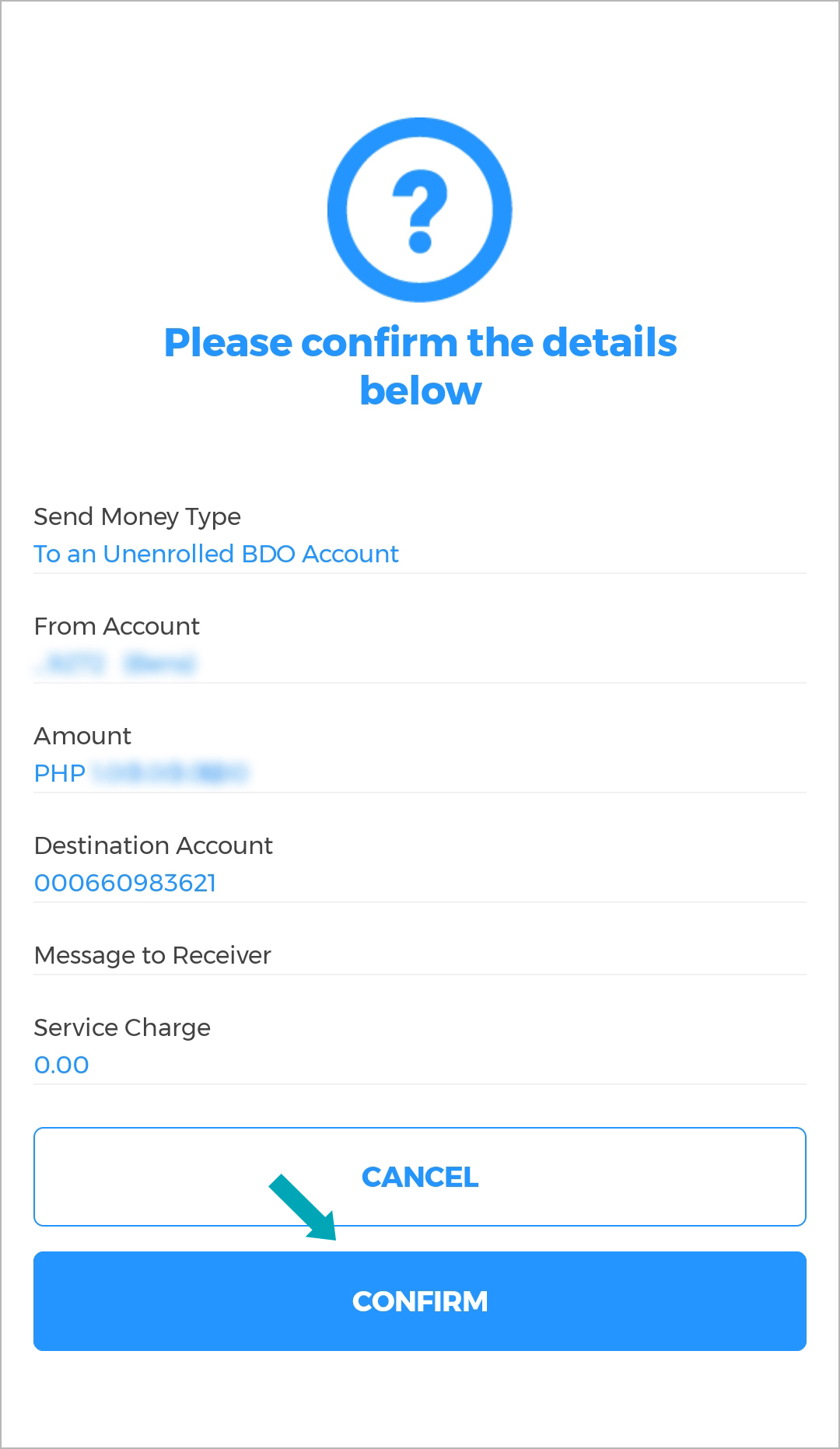The image is a screenshot from a mobile device interface, featuring a predominantly white background with a thin gray border surrounding the edges. At the top-center of the screenshot is a thick, baby blue circle containing a bold question mark. Below this, in bold blue text, the words "Please confirm the details below" are prominently displayed. 

The first section lists "Send Money Type" accompanied by a blue hyperlink reading "To an unenrolled BDO account," where the first letter of each word is capitalized except for "an," and "BDO" is in all caps. Next, the section labeled "From Account" shows blue text that is blurred and pixelated, obscuring the details.

Following this is the "Amount" section, indicating the currency in capital letters "PHP," with further blue text that is also blurred and pixelated. Beneath this is the "Destination Account" section, displaying the number "000-6609-83621." The "Message to Receiver" section follows, and at the bottom, "Service Charge 0.00" is indicated.

At the bottom of the screenshot, there are two buttons: a "Cancel" button and a prominent blue "Confirm" button with a right-facing arrow pointing towards it.